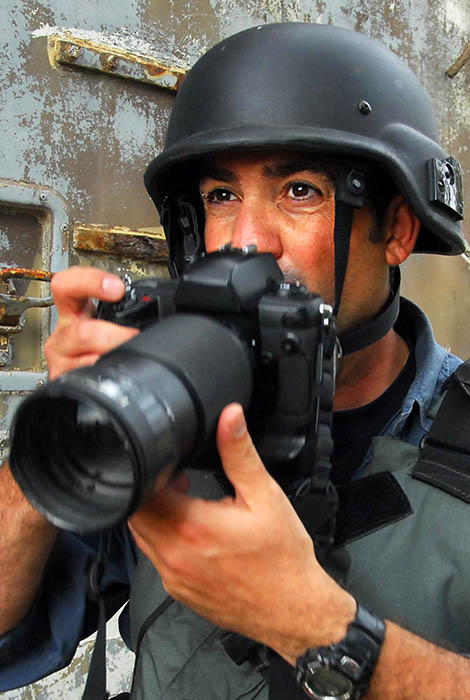A detailed image shows a war correspondent, identifiable by his large black military helmet adorned with an indiscernible decal on the side, and a protective vest that appears green or gray. He stands under broad daylight, with sunlight casting shadows on his gear. His gaze is directed towards the left, looking at something in the distance. In his hands, he holds a substantial black camera with a telephoto lens, poised as though he is ready to capture a moment. His right hand is on the shutter button, while his left supports the camera's base. A large wristwatch adorns his left wrist. His attire includes a black shirt under his vest and possibly a denim jacket. The background features an old, rusted metal structure, possibly the side or door of an armored vehicle, once painted light blue but now heavily worn and corroded. Despite the heavy gear, his posture is alert and focused, embodying the tense atmosphere of a war zone.